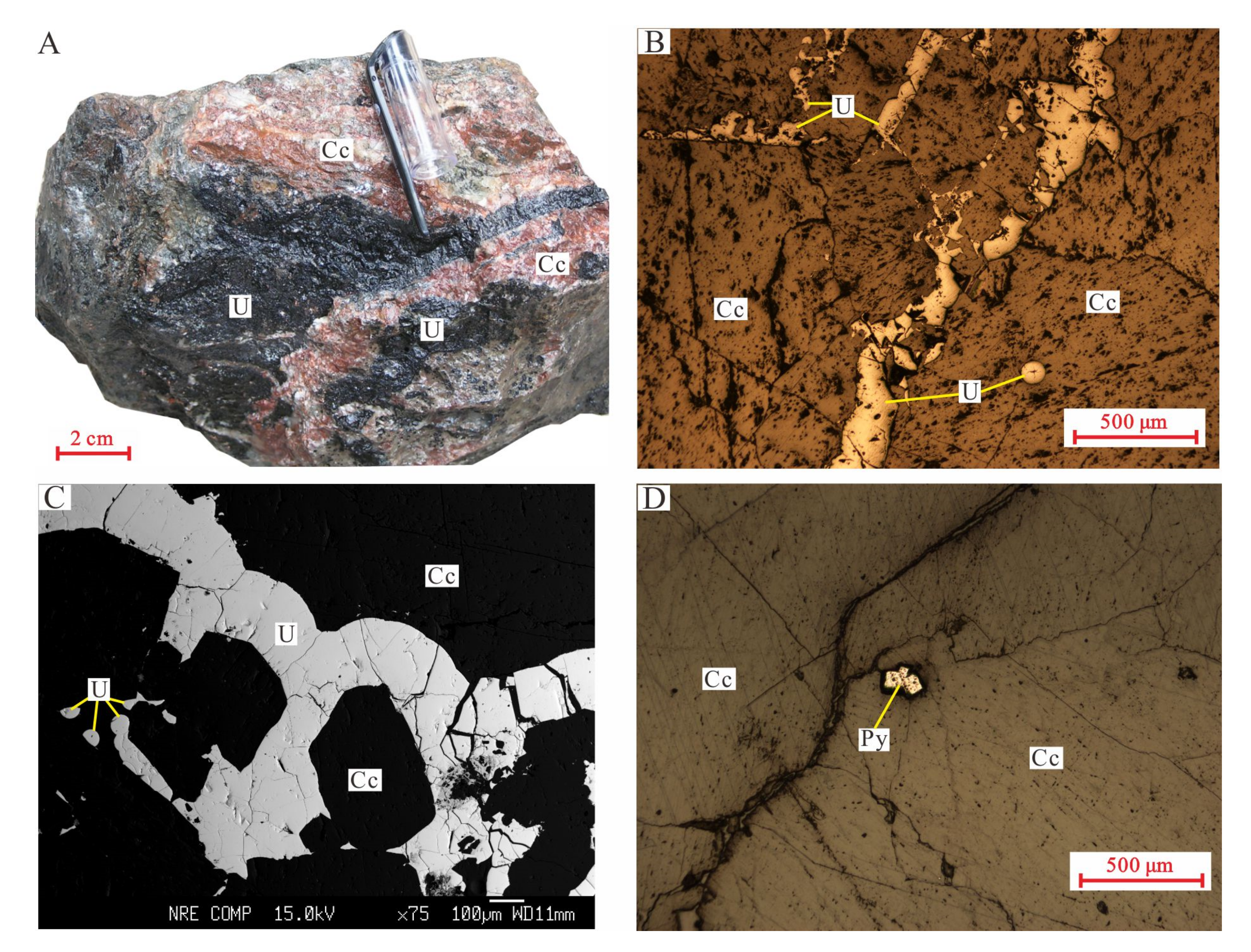The illustration consists of four images divided into two rows and two columns, labeled A, B, C, and D. Image A, located in the top left, displays a multicolored rock predominantly featuring black, red, and gray hues. A test tube or pen cover rests atop this rock. Visible on the rock are various letters and numbers, including "C-C-U," "2 cm," and "500 μm." To the right, Image B is a primarily brown illustration with some black and tan spots, accompanied by labels such as "C-C-U" and "500 μm." Moving to the bottom left, Image C showcases a black and gray mixture with markings that include "N-R-E COMP 15-O-K-V" as well as repeated "CC" and "UU" in different areas. Finally, Image D on the bottom right presents a darker brown and black surface with gold spots in the center, also marked with "CC" and "Pγ," as well as a scale indicating "500 μm."